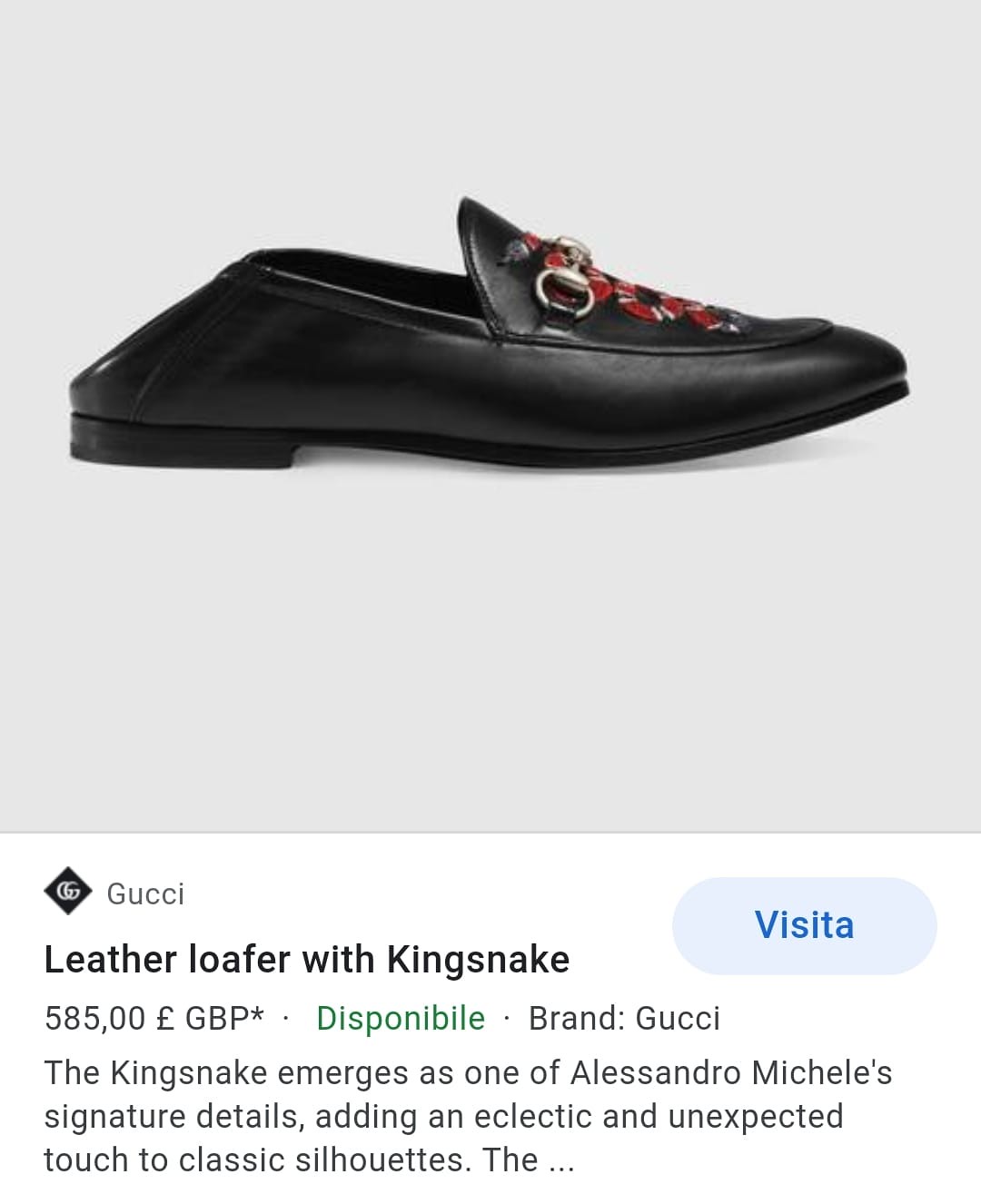The image features a sophisticated black leather loafer from the luxury brand Gucci, known as the "Leather Loafer with Kingsnake." Designed by Alessandro Michele, the loafer showcases a distinctive Kingsnake motif, one of his signature details that adds an eclectic and unexpected touch to the classic silhouette. The loafer's front is adorned with a silver ring and vertically aligned red accents. It appears that the back of the shoe is open, enhancing its unique design. The image, likely sourced from an internet browsing search result, displays the Gucci logo and product information below the shoe, listing the price at 585,000 GBP. A light blue clickable button labeled "Visita," which translates to "Visit," offers a link to further engage with the product.